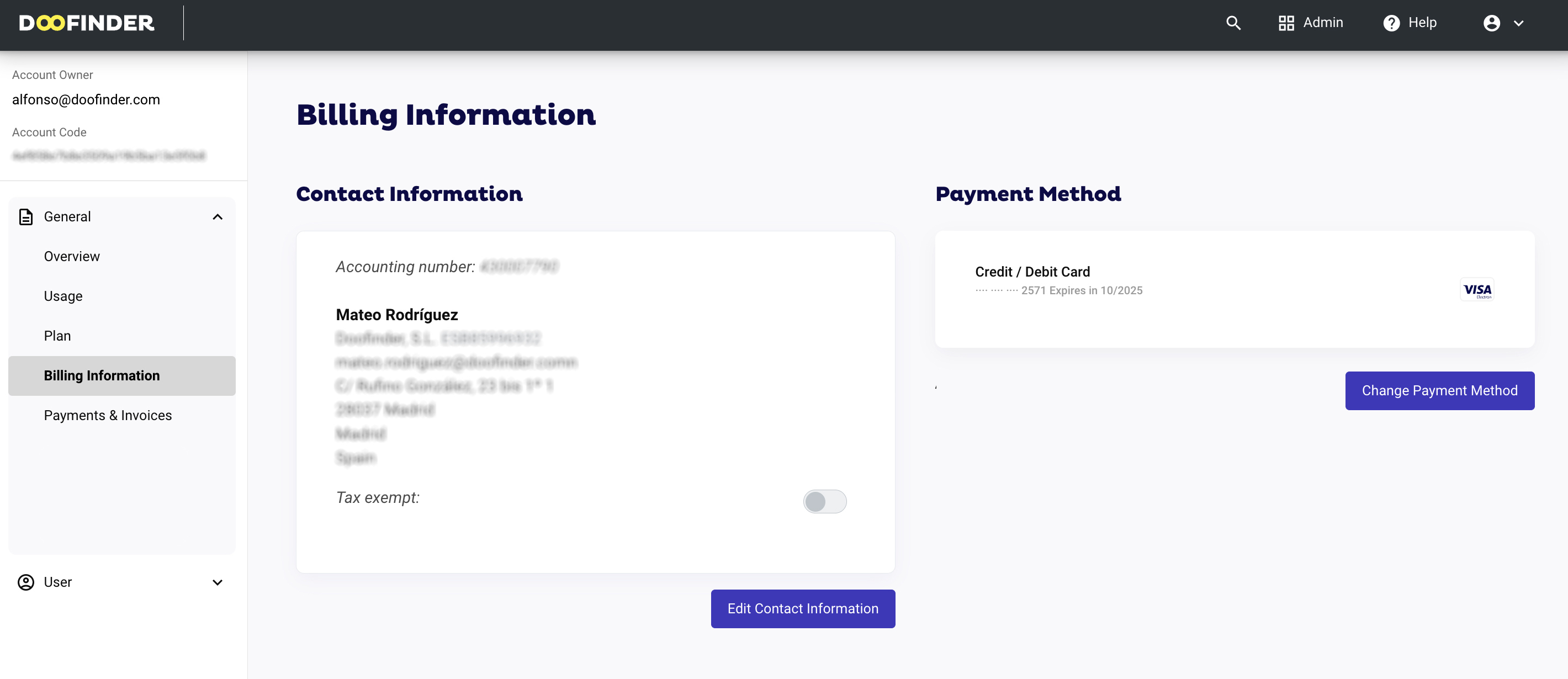This detailed screenshot from the DoFinder website highlights various aspects of the account owner's page. In the top left corner, the account owner's email is visible, while other personal details, including the account number and address, are blurred for privacy. The central focus of the screenshot is the billing information, where the details of a linked Visa credit/debit card are partially obscured, revealing only the last four digits and the expiry date of October 2025. Additionally, the tax exemption status indicates that Mateo Rodriguez is not tax-exempt.

The user interface includes several navigational options. The top right corner features administrative shortcuts such as 'admin,' 'help,' and 'more account information,' alongside a search bar for easy access. On the left side, a menu lists various sections: 'general,' 'overview,' 'usage,' 'plan,' 'billing information,' 'payments and invoices,' and a user dropdown menu. Notably, there are purple clickable labels for editing contact information and changing the payment method, streamlining user experience and accessibility.